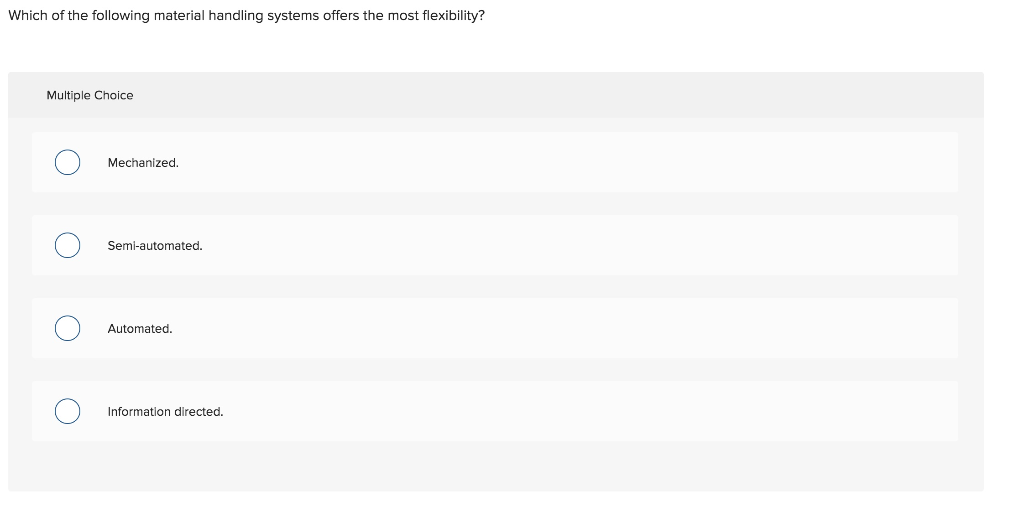This landscape-oriented photograph features a multiple-choice question set against a predominantly white background with a central gray box. Positioned at the top left, black text poses the question: "Which of the following material handling systems offers the most flexibility?" Directly beneath, a darker gray header labeled "Multiple Choice" introduces four rectangular white boxes, each representing a possible answer. To the left of each box is a bubble followed by the corresponding choice in black font. The answers presented are: 1) Merchandise, 2) Semi-automated, 3) Automated, and 4) Information directed. This question seems to be part of a test, likely associated with logistics, automated factory operations, or a related professional field, aimed at assessing knowledge on material handling systems.